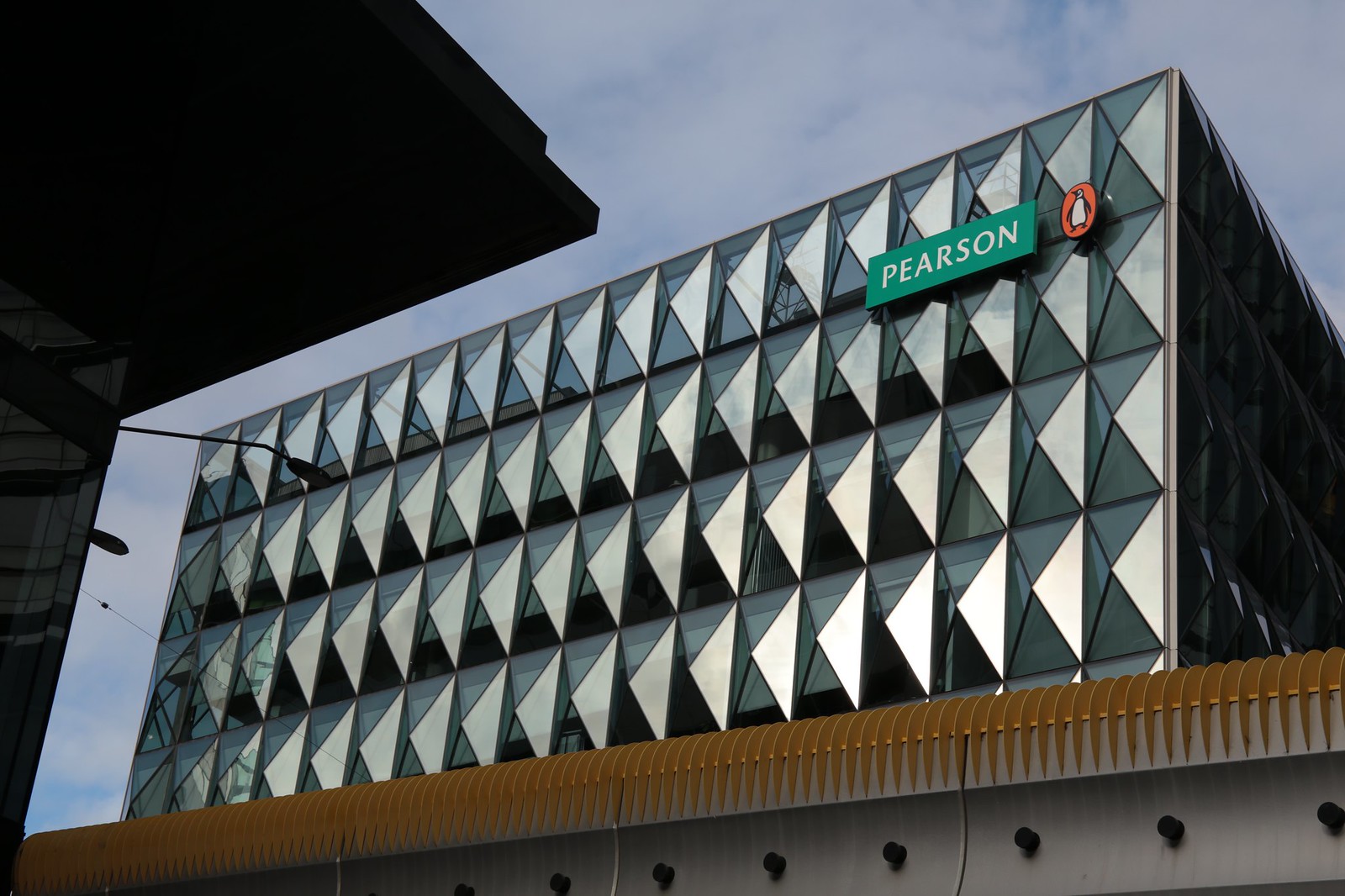The image depicts an upward perspective of a striking architectural scene featuring a large square glass building adorned with a patterned texture of protruding triangles, resembling almost flat pyramids. The building’s surface, interspersed with white and black windows, creates a diamond-like appearance due to the interplay of sunlight and shadow. In the top right corner of the building, a green rectangular sign with the word "Pearson" in white font stands out, adjacent to an oval emblem showcasing an illustration of a penguin with a white front and black limbs on an orange background. Surrounding the building, the background reveals a clear blue sky dotted with white clouds, enhancing the visual depth. In the lower portion of the image, a distinctive object stretches horizontally from the left to the right side, featuring a yellow top, white sides and bottom, and black bolts running through it. This object is situated against what appears to be a concrete walkway characterized by a series of oval, arch-like grid marks, further adding to the complexity of the scene.